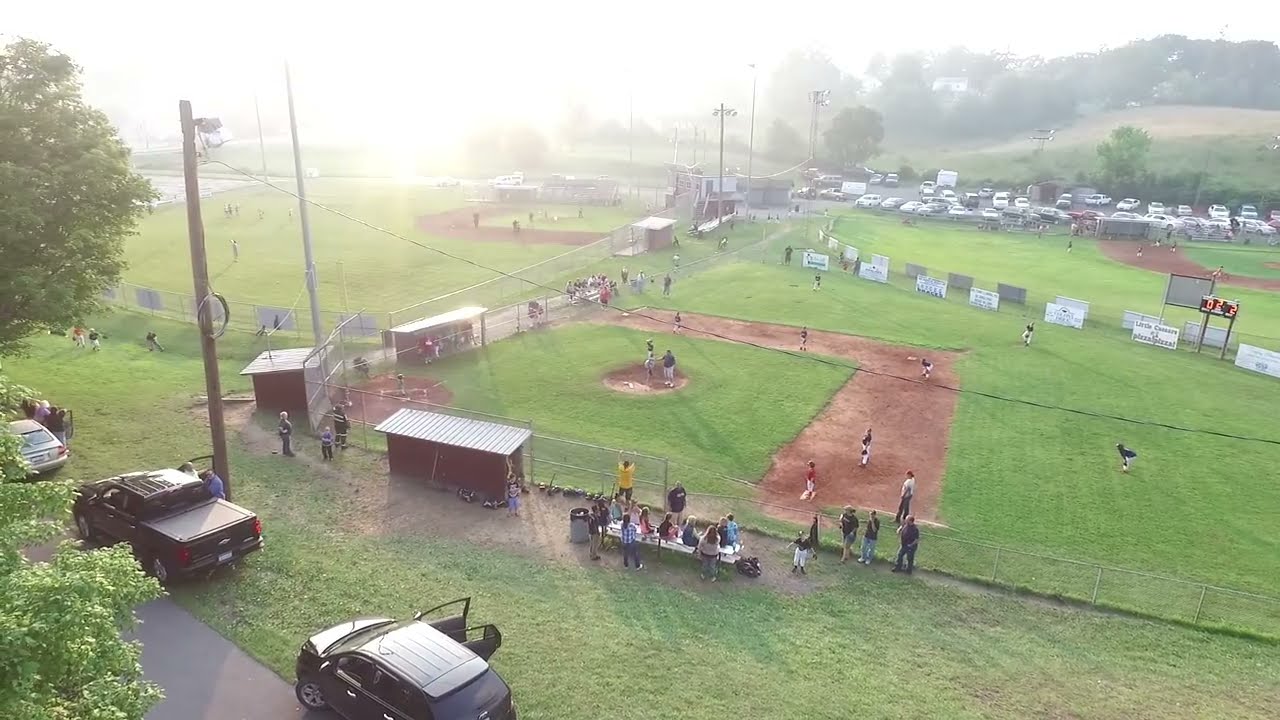The image captures an elevated view of a vibrant baseball scene, seemingly taken from one or two stories up in a tower or building. In the foreground, a game is actively in progress on a baseball diamond made of dirt and grass, marked by bright sunlight in the top left corner that casts an intense glare across the image, partially washing out some details. Players in blue and red uniforms and helmets are situated around the field, with a small scoreboard showing double twos, hinting at an ongoing competitive game. Surrounding the main field is a silver metal railing with benches and seating occupied by spectators, both adults and children, eagerly watching the action. In the vicinity, team members sit on the bench waiting for their turns to play. 

Beyond the primary field, the expansive grassy area features at least two other baseball diamonds, one positioned in the upper left and another in the upper right of the image, each fenced off with dividers to keep the games from overlapping. All diamonds are bustling with activity. In the background, a fully packed large parking lot stretches in the top right corner. Additionally, a small parking area is visible with a mix of vehicles, including cars parked with their doors open for unclear reasons. Nearby, more cars, including a pickup truck and a small hatchback, are parked along a road in the left foreground. The setting sun not only illuminates the scene but also adds a dramatic, almost ethereal quality to the photograph. The photo comprehensively encapsulates the lively, community-centric atmosphere of a local baseball event during sunset.